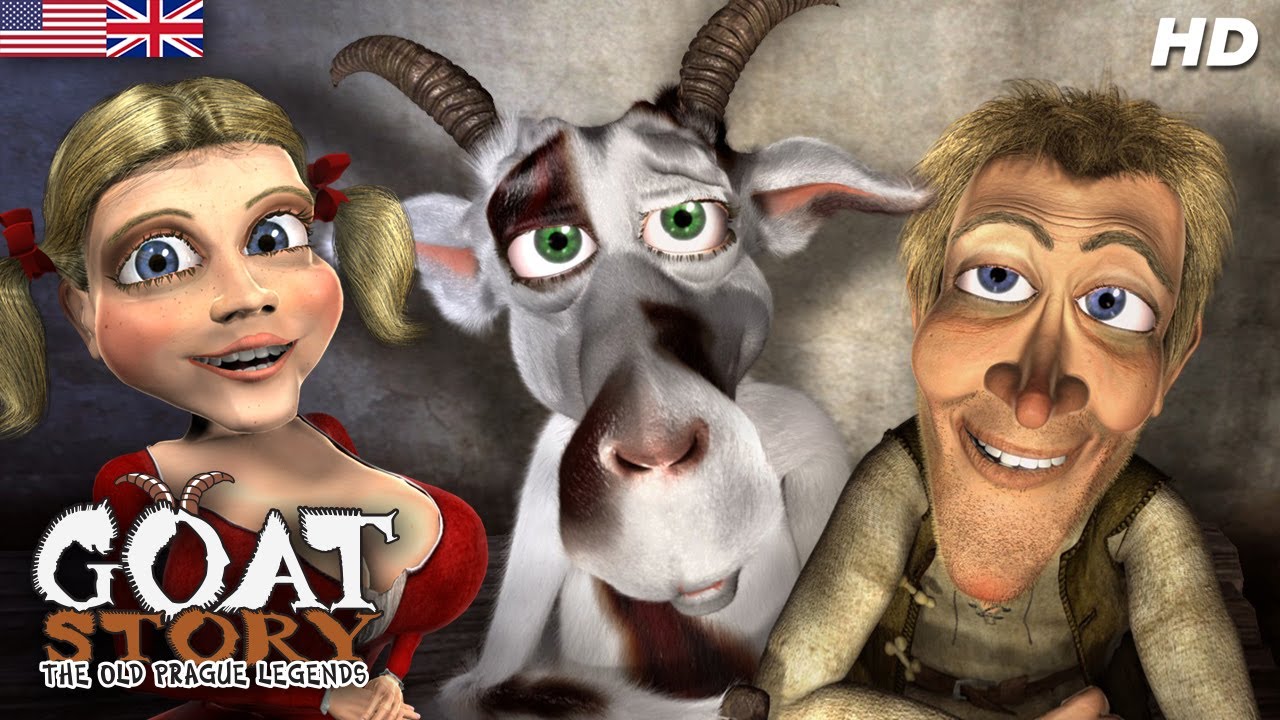This highly detailed photograph appears to be an advertisement for a game titled "Goat Story: The Old Prague Legends." In the top left corner, the American and British flags are prominently displayed, while the top right corner features the "HD" logo, indicating high definition quality. Dominating the center of the image are three characters: a woman, a goat, and a man. 

The woman, positioned on the left, has striking blonde hair styled in pigtails adorned with red bows. She has blue eyes and wears a revealing red top that highlights her large bosom. In the middle stands the goat, distinguished by its green eyes. The goat's predominantly white fur is accented by patches of brown, including a significant patch over one eye, on part of its nose, and on its chest. It also features two dark brown horns, pink and gray ears, and a gray and brown nose and mouth. 

On the right side is a man, who also has blue eyes, although one appears slightly lazy, giving him a tired look. His short blonde hair and peasant-style clothing in muted, grayish-brown colors suggest a rustic background.

In the bottom left corner, the title "Goat Story" is written in a hairy font with horn-like embellishments on the letter "O." Directly below it, in brown, is the subtitle "The Old Prague Legends." This detailed composition places emphasis on the main characters while ensuring all significant text and graphical elements are clearly noted.